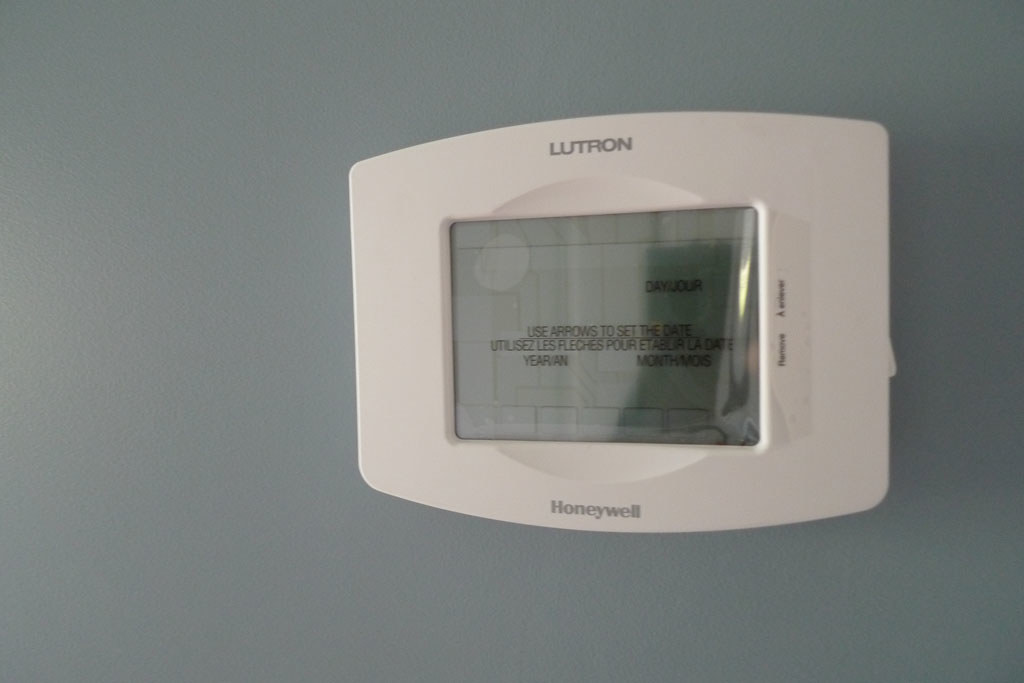A freshly installed, sleek Honeywell thermostat adorns a modern wall painted in a sophisticated blue-gray hue. This new addition, still wrapped in protective plastic over its screen, indicates recent installation—likely in a newly built home or one about to hit the market. The square, white thermostat displays instructions in both English and French, prompting users to use arrows to set the date. The absence of physical buttons suggests a contemporary, touchscreen interface, aligning perfectly with the modern aesthetic of the space. The wall’s color, a blend of blue with gray tones, contributes to the overall modern and trendy feel, indicative of current design trends in new constructions.